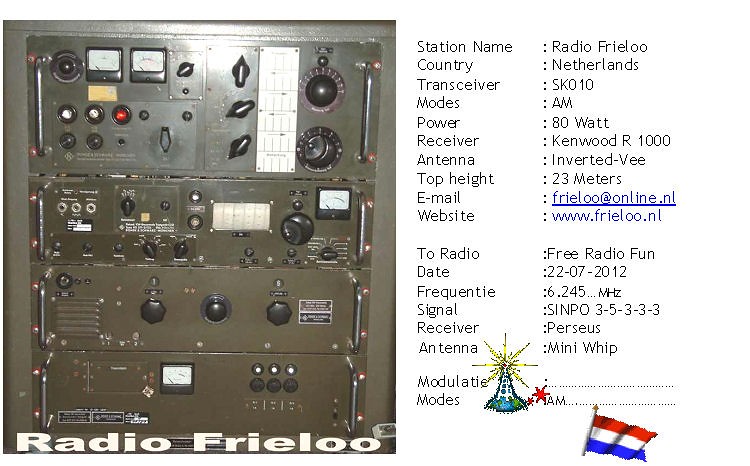The image features the front panel of a brownish-green radio transmitter, likely designed for aviation or similar technical use. The left side is divided into four sections with numerous black knobs, dials, gauges with white backgrounds, and metallic silver handles on the outside. Some panels appear to contain operating instructions or dynamic information. Notably, one of these sections is labeled with "radio, free lube" in white text.

On the right side of the image, detailed informative text lists several specifications:
- Station Name: Radio Free Lube
- Country: Netherlands
- Transceiver: SK010
- Modes: AM
- Power: 80 watts
- Receiver: Kenwood R1100
- Antenna Top Height: 23 meters
- Email: freelue@online.nl
- Website: www.freelue.nl

Additional details include transmission data such as frequency (6.245 MHz), signal strength (SINPO 3-5-3-3-3), receiver (Perseus), and antenna type (mini whip). Underneath the detailed text, it states "modulate modes: AM."

Central to the image is an illustration of a radio antenna emitting yellow streaks of light in all directions, accompanied by red stars. At the bottom of the image, a Dutch flag, comprising red, white, and blue horizontal stripes, is depicted waving on a slightly tilted silver pole capped with an orange tip.